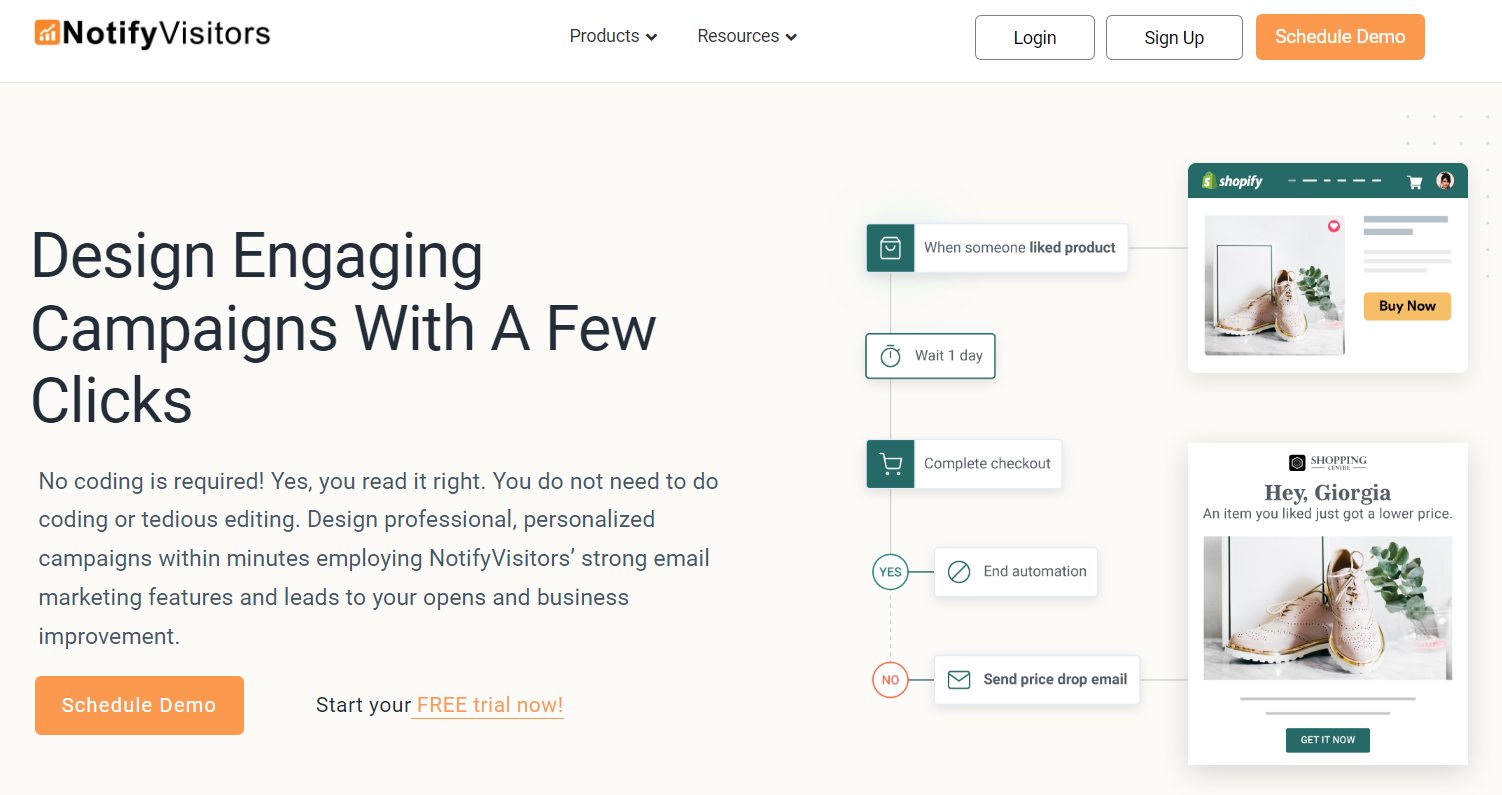In this image, we see a screenshot of a web interface designed for a marketing tool. In the upper left corner, black text reads "Notify Visitors" accompanied by a logo to its left. Next to this, there is an orange box with white print. To the right of this, there are dropdown menus labeled "Products" and "Resources," in addition to two white buttons. Further to the right, there are options to "Log In" and "Sign Up," followed by an orange button labeled "Schedule Demo."

Beneath this navigation bar, there is a large bold black text that states, "Design engaging campaigns with a few clicks. No coding is required. Yes, you read it right. You do not need to do coding or tedious editing." The text emphasizes that users can design professional, personalized campaigns within minutes using the robust email marketing features offered by Notify Visitors, aiming to enhance open rates and overall business improvement.

At the bottom of the visible section, there is a yellow action button labeled "Schedule Demo."